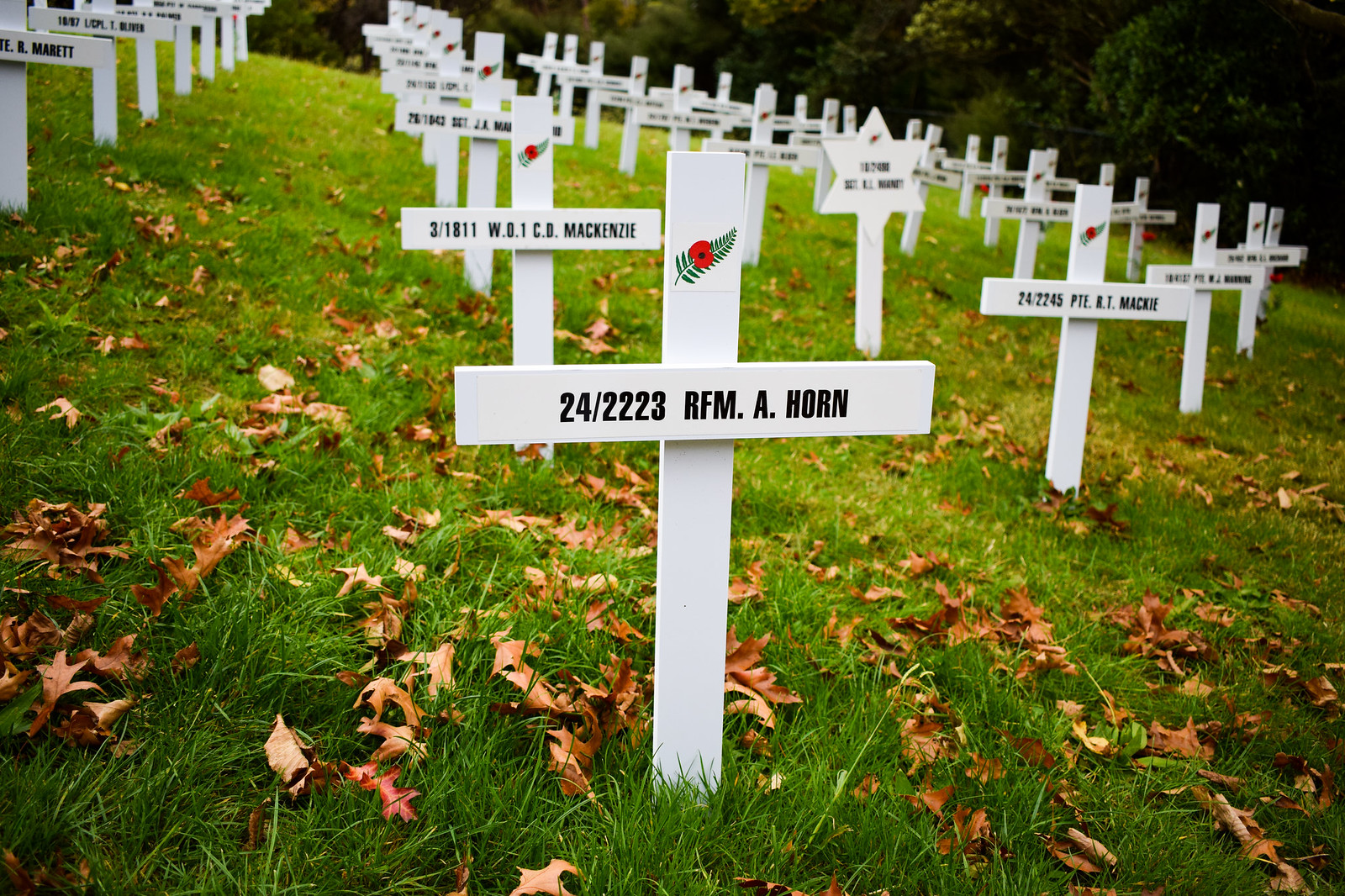The image is a photorealistic close-up of a cemetery with long rows of white crosses standing in bright green grass scattered with brown and red leaves. The central cross, prominently featured in the middle of the image, bears the inscription "24/2223 RFMA." At the top of this cross, there is a sticker with a long green leaf and a red poppy. Behind this central cross, another row of white crosses with various names written in black text stretches into the distance, extending to the left and right, creating a sense of depth and multitude. Additionally, there appears to be a single star-shaped headstone among the crosses. In the background, the scene is framed by dense copses of vibrant green trees, adding to the solemnity and tranquility of the setting.